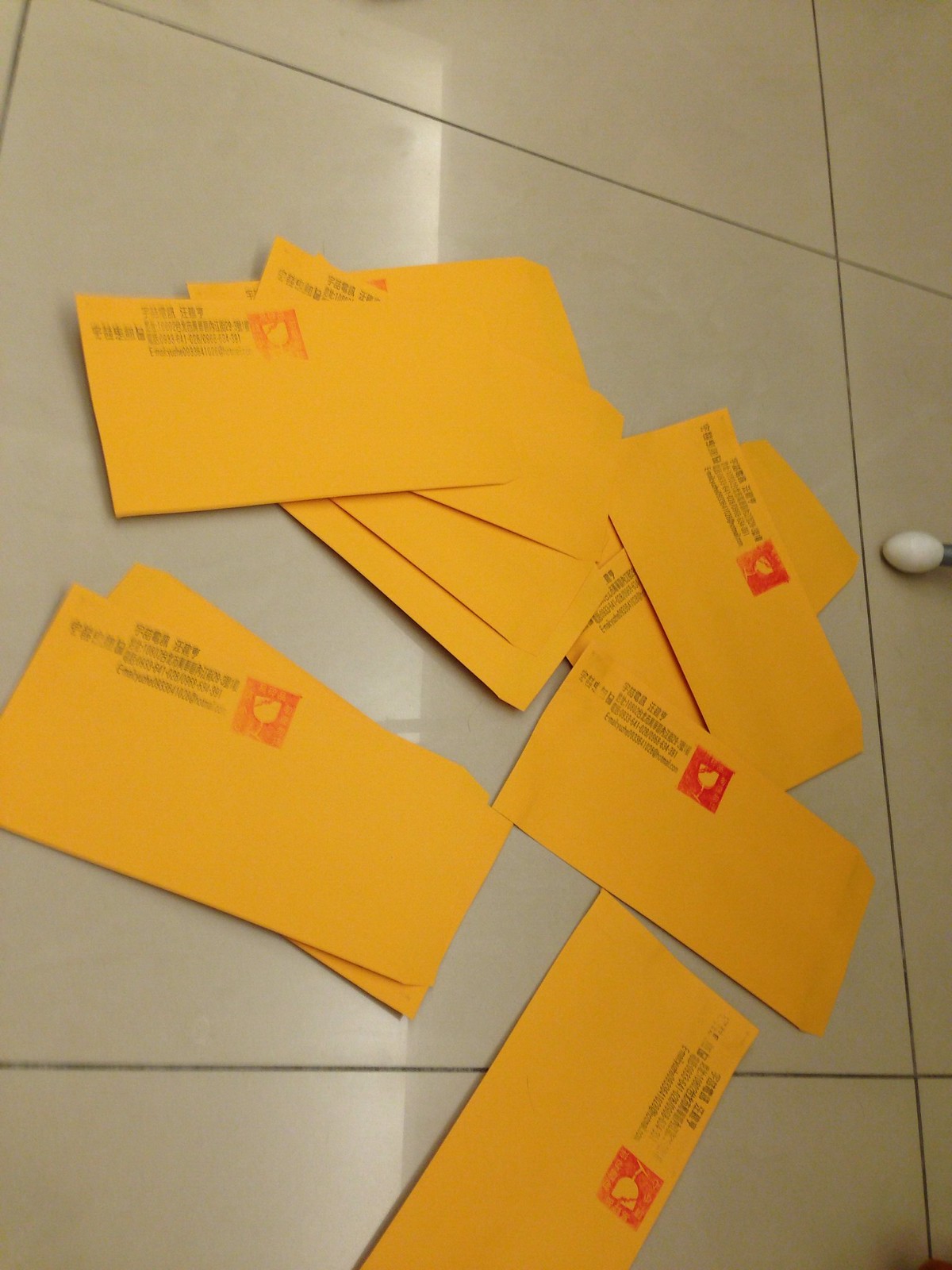The image captures a vertically oriented, overhead view of a glossy tan tile floor with large square tiles separated by darker lines. The reflective surface of the floor shows a white overhead fluorescent light and casts shadows. Scattered across this floor is a pile of long, business-size envelopes in a darker yellow hue, almost orange. Each envelope bears a return address in black text in the top left corner, alongside a red stamp featuring a chalice or wine glass framed by a border pattern. The envelopes appear randomly thrown yet somewhat stacked. In the center-right of the image, a white, plastic-tipped chair leg is visible.